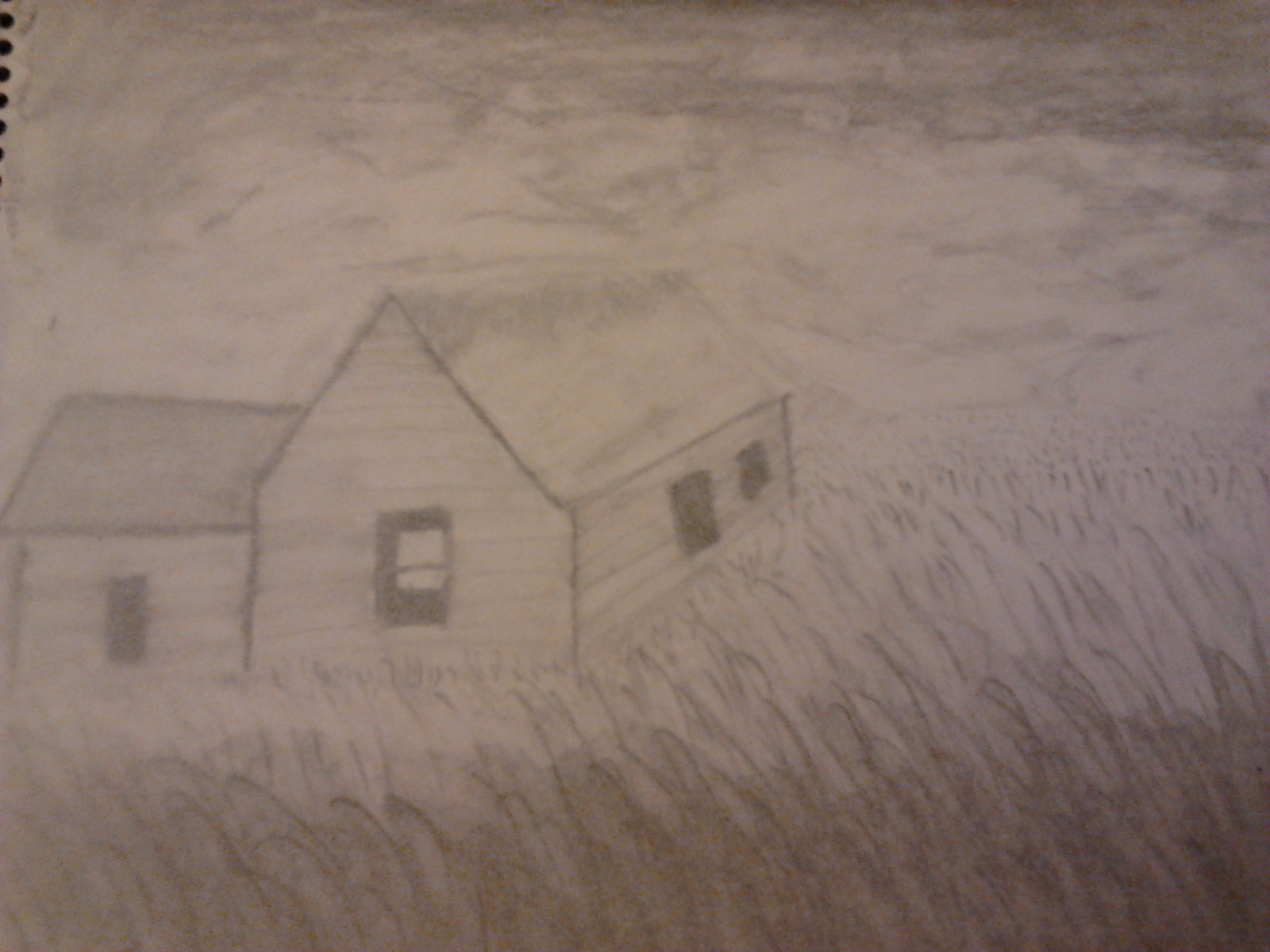A hand-drawn illustration in a spiral-bound notebook is depicted, with the faint black spirals visible in the upper left-hand corner. The drawing features a modest house with a triangular roof and a rectangular overhang. The right side of the house showcases two darkly-shaded windows, likely sketched with a pencil or gray medium. The front of the house has another window providing a hint of interior dimension through a lighter white area. An extension on the left side of the house includes a second, darker roof, wall structures, and a door. Surrounding the house is an abundance of grass or weeds, implying a field or untended garden. The background reveals a gray sky dotted with puffy white clouds, adding depth to the scene.